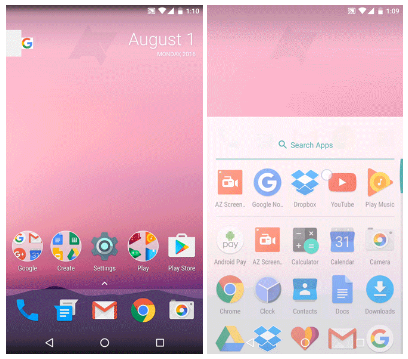The image consists of two side-by-side screenshots of a phone's home screen, set against a vibrant background with an ombre effect of various shades of pink, transitioning to a rich dark magenta at the bottom.

On the left-hand screenshot, the familiar Google 'G' logo is prominently displayed at the top left. The time shown is 1:10, and the date is August 1st, Monday, presumably from the year 2018. This screen indicates a battery level slightly more than half, alongside white Wi-Fi and cellular reception icons.

The home screen features two rows of icons. The first row of icons includes 'Google,' 'Create,' 'Settings,' 'Play,' and 'Play Store.' The second row contains a blue phone icon, a messaging app with one blue and one white text box, the Gmail symbol, the Google app, and Google Photos.

The right-hand screenshot displays a different part of the phone's interface, showing a pop-up with 20 icons. The time shown here is 1:09, with the battery, Wi-Fi, and reception icons identical to those on the left screen, albeit without a visible date. The icons in the pop-up include 'AC Screen,' 'Google,' 'Old (presumably an app shortcut),' 'Dropbox,' 'YouTube,' and 'Play Music.' Following these are 'Android,' 'Play,' 'Easy Screen,' 'Calculator,' 'Calendar,' 'Camera,' 'Chrome,' 'Clock,' 'Contacts,' 'Docs,' and 'Downloads.' Due to the zoom level, the last row of icons is cut off, making them unreadable.